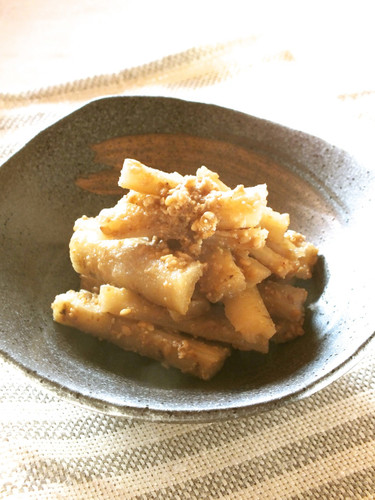A close-up image showcases a handmade, square-shaped brown ceramic bowl with rounded edges, set atop a linen tablecloth or placemat featuring gray and white stripes. The bowl is filled with a pile of fried pasta, resembling either penne or rigatoni, with a golden, deep-fried crust encasing it. The pasta appears to be layered in about four distinct tiers. A combination of grated cheese and perhaps nuts or butter generously coats the dish. The lighting, coming from the upper right, floods the scene with bright white light, causing parts of the bowl to wash out and merge with the blurred white background, adding to the rustic yet vibrant presentation.